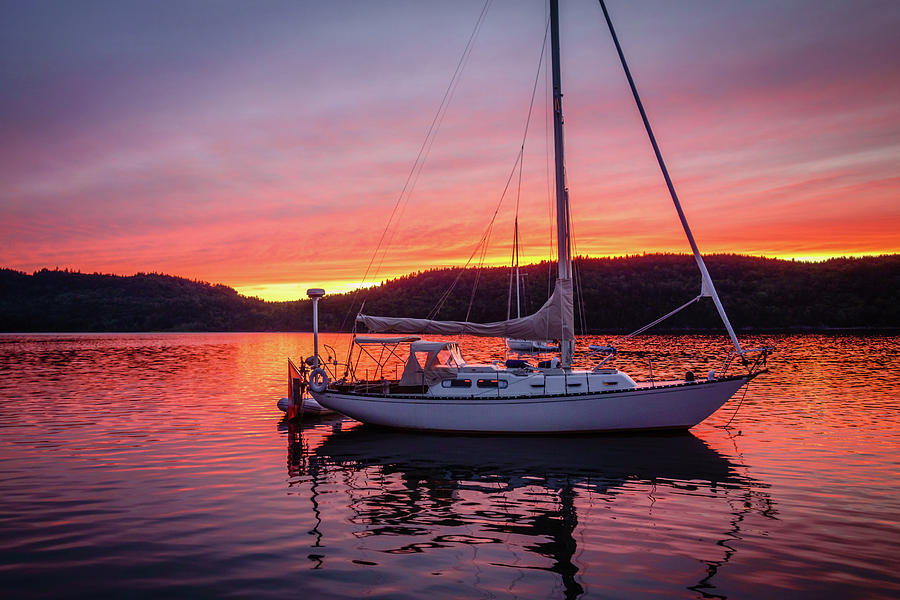A professionally taken photograph captures a tranquil sunset scene on a calm lake, framed by large grassy hills partially blocking the setting sun, whose golden and orange light peeks out, casting a serene glow over the water. The unmoving, modern white sailboat, with its sails retracted, is centered prominently in the image, appearing completely dormant. Reflections of the sunset's oranges, yellows, and purples play off the rippling water, adding a painterly quality to the scene. The background reveals a forested horizon, enhancing the scenic, picturesque atmosphere. Absent of any people or text, this high-quality image conveys a peaceful and moodily lit lakeside moment.